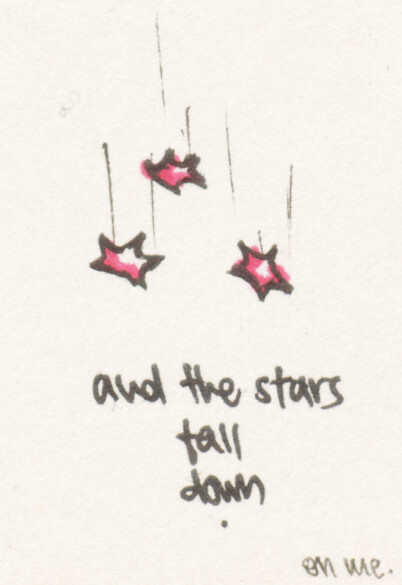The image features a minimalist drawing on a white background, composed primarily with black and pink markers. Six thin, vertical black lines descend as if tethering onto three stars, giving the illusion that the stars are falling or being suspended on strands. Each star is outlined in thick black marker, with partial fills of vibrant pink and patches of white paper showing through, suggesting a spontaneous, youthful touch akin to a child's or teenager's artwork. At the bottom of the image, the phrase "And the stars fall down" is inscribed, with "Fall" uniquely in cursive and the rest in printed letters. Below this text, a solitary black dot is placed, hinting at a possible correction or artistic detail. The image is signed in the bottom right corner, though the signature is faint and difficult to decipher.